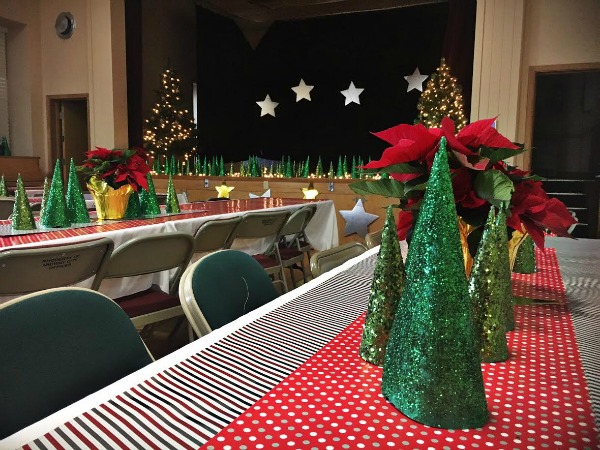This interior photograph captures a detailed close-up of a long table set up in an auditorium, meticulously decorated for a Christmas event. The table is covered with a red and green striped tablecloth, adorned with a middle runner featuring yellow, green, and white polka dots. Positioned centrally on the table is a glittering green cone tree centerpiece, accompanied by golden pots holding vibrant poinsettias. The background reveals a stage with a black curtain embellished with four silver stars, flanked by smaller, shimmering green cone trees aligning the front. Numerous folding chairs, some draped with green fabric, surround the table, suggesting an awaiting banquet. Additional features include lit Christmas trees at the stage corners, enhancing the festive atmosphere. The overall scene, devoid of people, hints that the event is about to commence, ready to host a joyous Christmas gathering.